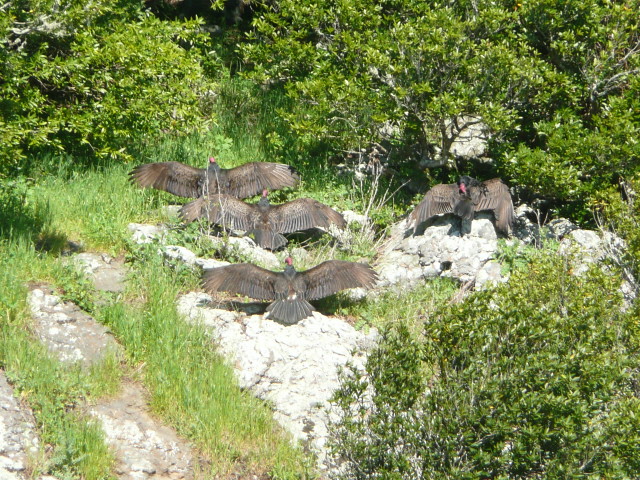The photograph captures a serene nature scene featuring four birds, likely vultures, with striking bright red heads and dark brown feathers, some appearing black due to lighting variations. These birds are grounded on an area interspersed with light gray rocks, patches of green grass, and a few leafy green bushes. Each bird exhibits its wings outstretched, highlighting an impressive wingspan, though one on the right is only slightly spreading its wings, possibly engaged in grooming. The birds' arrangement forms a rough T-shape: two positioned in the back, with one each on the upper left and upper right, another bird stands to the lower right, slightly off to the side perched on a rock, and one more bird, centrally placed, aligns itself with the others, creating a striking symmetry in the scene. The backdrop includes a mix of trees or shrubby greenery, enriching the natural ambiance of the setting.